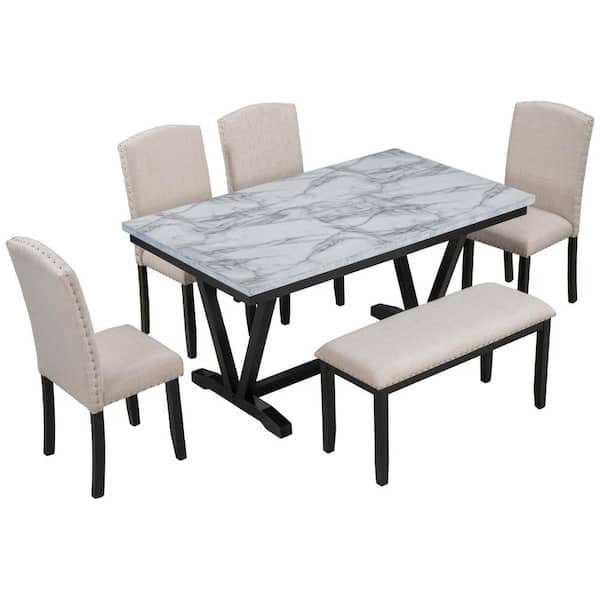The image showcases a modern dining room set against a white background. The central piece is a rectangle-shaped dining table with a marble-style tabletop and an intricate black support structure, featuring a V-shaped stand leading into a single stabilizing leg. Surrounding the table are four chairs and a bench, all sharing a cohesive design. The chairs and bench feature sleek black frames with padded white seats, fastened by buttons, adding a touch of elegance. The long side of the table on the left has two chairs, while the bench without a backrest spans the right side of the table, accommodating the space of two chairs. Additionally, at each short end of the table is a single chair, making a total of four chairs and one bench. The clean lines and monochromatic color scheme create a sophisticated and inviting dining area.